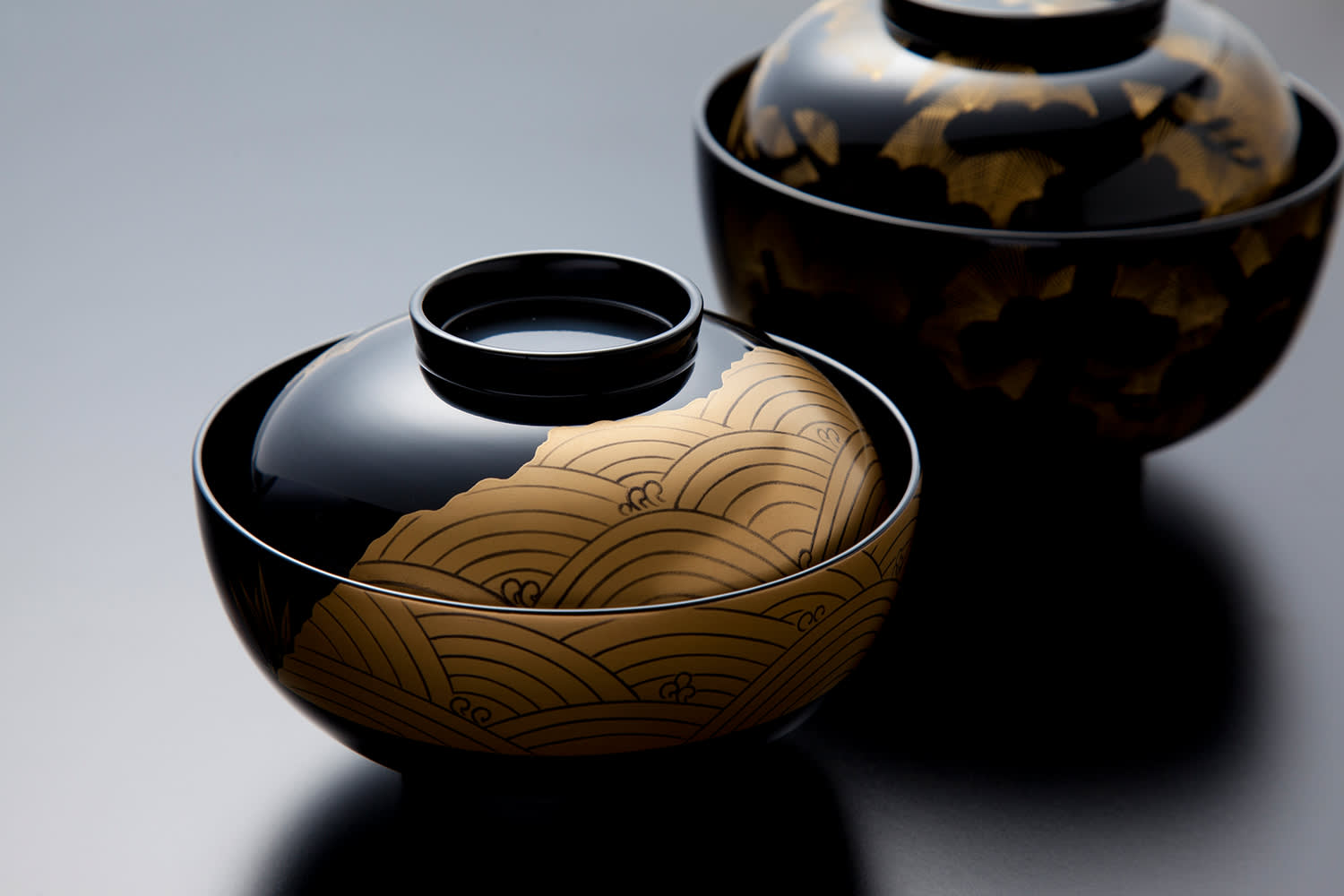This color photograph captures two intricately designed Japanese pottery bowls, made of black glazed ceramic. The foreground features a bowl adorned with a stylized black and gold wave print, illustrating a popular Japanese art motif with concentric, overlapping half circles. The design is reminiscent of rainbows with only black outlines, forming three rows around the bowl. The lid fits snugly, suggesting it could serve as a plate for rice or side dishes.

The background bowl, slightly askew and taller, showcases a black silhouette intricate with inlaid gold patterns depicting trees or possibly sakura blossoms. Despite both bowls having visible shadows, they are placed on an empty, digitally removed, white or gray background typical for product photography. This detailed scene highlights the artistry and functional design of these Japanese ceramic pieces, potentially aimed at a consumer market.